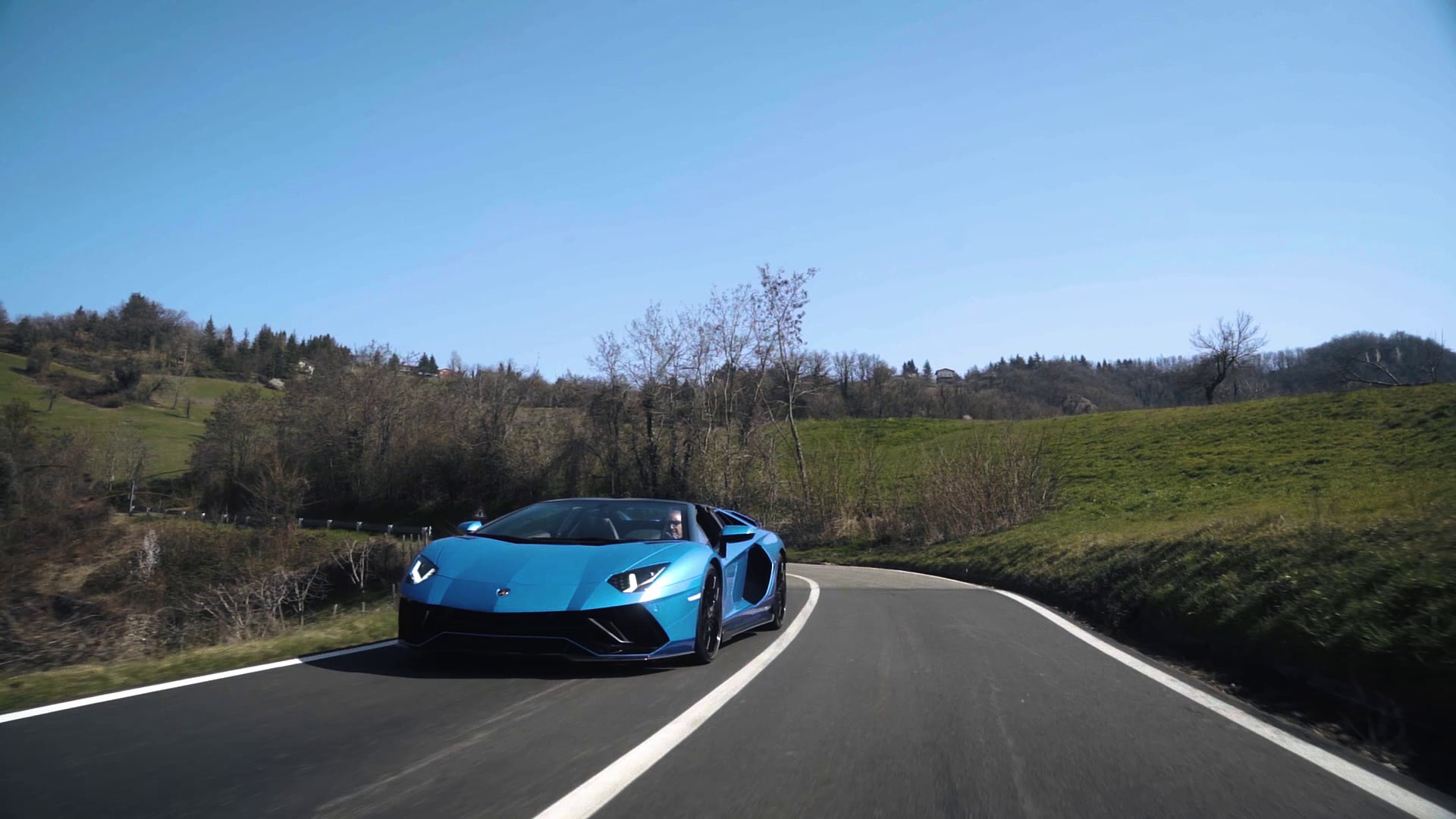In this picturesque scene, a sleek, light blue Lamborghini with black trim and wheels drives down a winding, gray asphalt road, which features white lines on its edges and a solid white stripe down the center. The road, situated in a rural countryside setting, is flanked by sparse greenery and grass patches. Behind the car, a ridge line of trees stretches across the horizon, transitioning into rolling hills that hint at a season possibly late fall or winter, with the trees appearing somewhat barren. A clear, blue sky, gradually lightening towards the horizon, occupies the upper half of the image, adding depth to the serene backdrop. The Lamborghini, driven by a man visible through the window, appears in motion, enhancing the dynamic feel of this tranquil countryside drive.